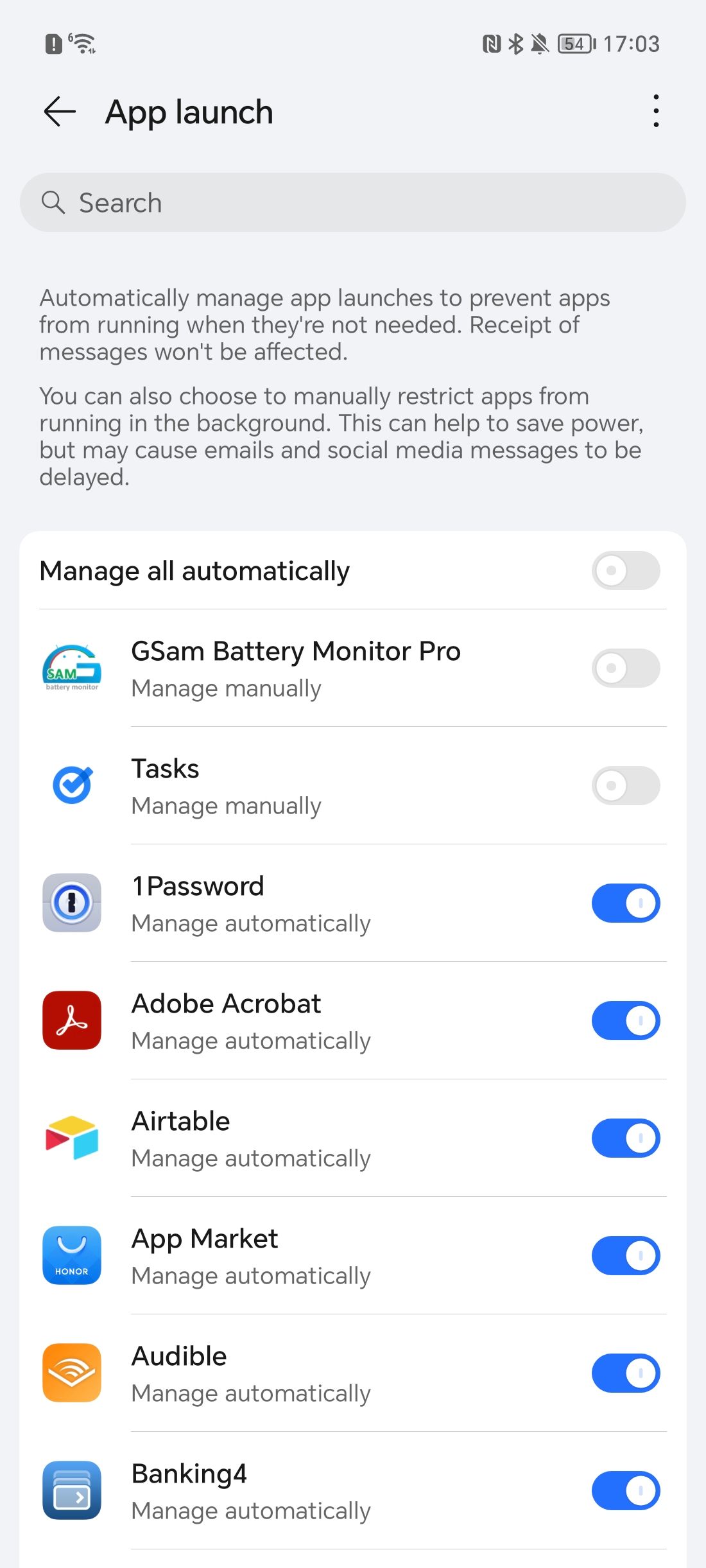This detailed descriptive caption accompanies a screenshot taken from a cell phone.

At the very top of the screenshot, the device’s status bar is visible, indicating it is 5:03 PM (1703 in 24-hour format). The battery level is at 54%, and Bluetooth is enabled. An icon showing an alarm bell with a slash through it signifies that the phone is in silent mode.

The screenshot was taken within an application interface titled "App Launch." A back arrow is located to the left of this title, and to the right, there is a vertical stack of three dots representing the menu button. Below the title, there is a search box featuring a magnifying glass icon on its left and the text "Search."

The main section of the screenshot contains a heading "Manage All Automatically," under which is a list of installed apps with toggle switches next to them, allowing the user to manage these apps manually or automatically. The apps listed with their current management toggles are as follows:

1. GSAM Battery Monitor Pro - Toggle is off (managed manually)
2. Tasks - Toggle is off (managed manually)
3. 1Password - Toggle is on (managed automatically)
4. Adobe Acrobat - Toggle is on (managed automatically)
5. Airtable - Toggle is on (managed automatically)
6. AppMarket - Toggle is on (managed automatically)
7. Audible - Toggle is on (managed automatically)
8. Banking 4 - Toggle is on (managed automatically)

This comprehensive description captures the various elements visible in the cell phone screenshot, providing a clear understanding of its contents and context.